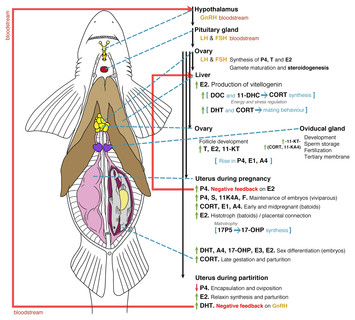This detailed diagram presents a cross-sectional view of a shark from the underside, showcasing various internal organs with clear labels and color highlights. The shark is depicted within a red-bordered outline, and there are dashed white lines pointing to detailed descriptions on the right side of the image.

Highlighted organs include the hypothalamus (marked within a small rectangle), the pituitary gland (situated between the gills and circled in red), and the prominently brown-colored liver that stretches over half the shark's body. Also depicted are the ovaries, oviducal gland, and uterus at different stages (pregnancy and parturition), all illustrated in distinct colors such as pink, purple, and yellow to differentiate between them.

The diagram features text annotations on the right, explaining the function and location of each organ. The visual representation suggests the shark may be pregnant, as smaller sharks are visible within the uterine area. The pencil-drawn illustration includes the shark's fins and distinctive features, like a rounded, pointed head without visible teeth.